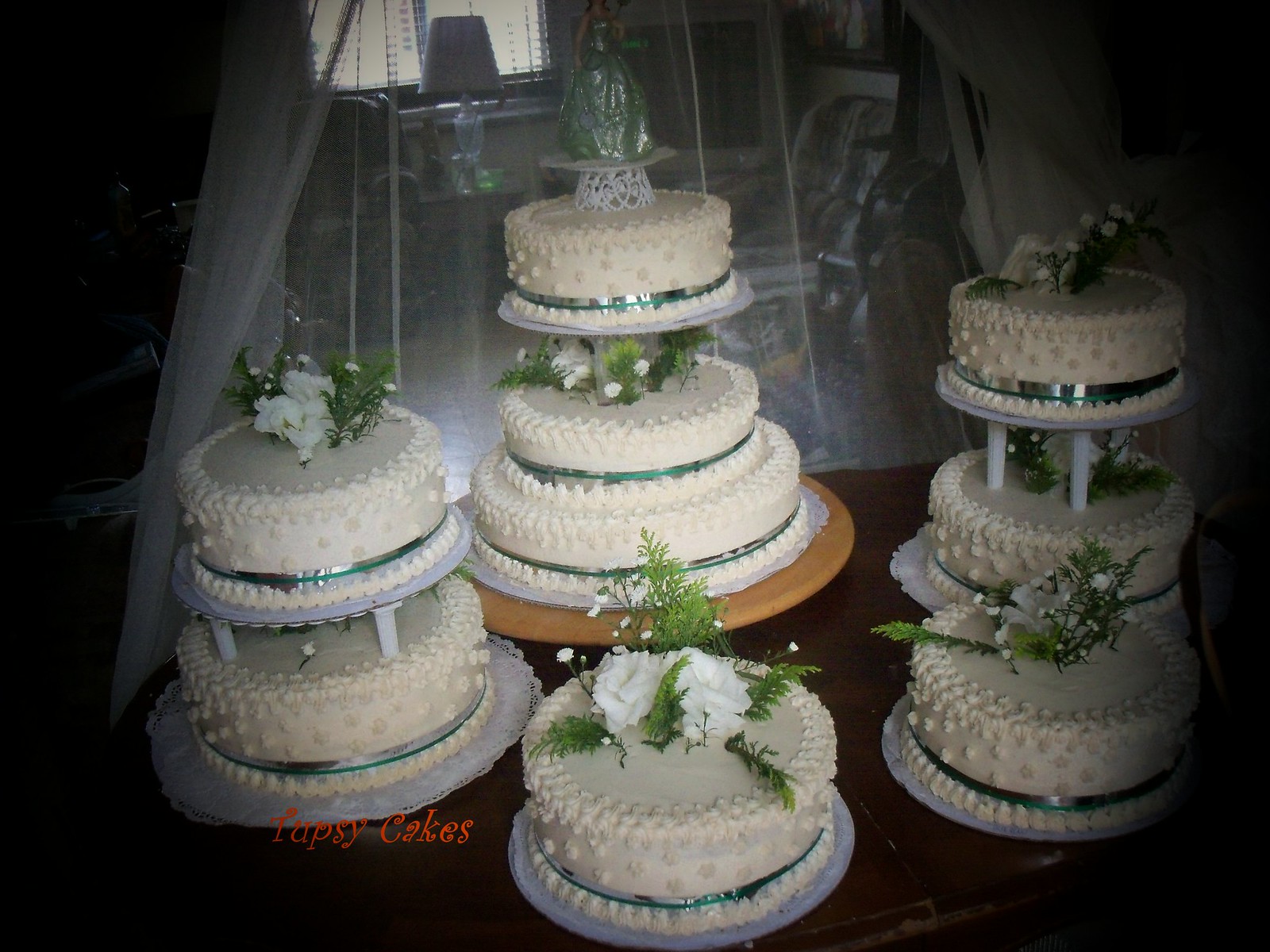This promotional image showcases an elegant display of five wedding cakes arranged on a dark wooden table in a home setting. The foreground is dominated by the cakes, each adorned with meticulous white frosting, delicate white flowers, and lush green leaves. Two of the cakes are single-tier, two are two-tier, and the centerpiece is a three-tier cake crowned with a sophisticated glass or acrylic figure. They're uniformly decorated with thin green bands encircling each layer, adding a touch of elegance. In the lower left corner, the text "Topsy Cakes" is prominently displayed in red. Draped behind the table is a sheer white fabric, through which an inviting living room is visible, complete with an upholstered chair, an end table with a lamp, and a window adorned with blinds, enhancing the cozy and intimate atmosphere of the scene.